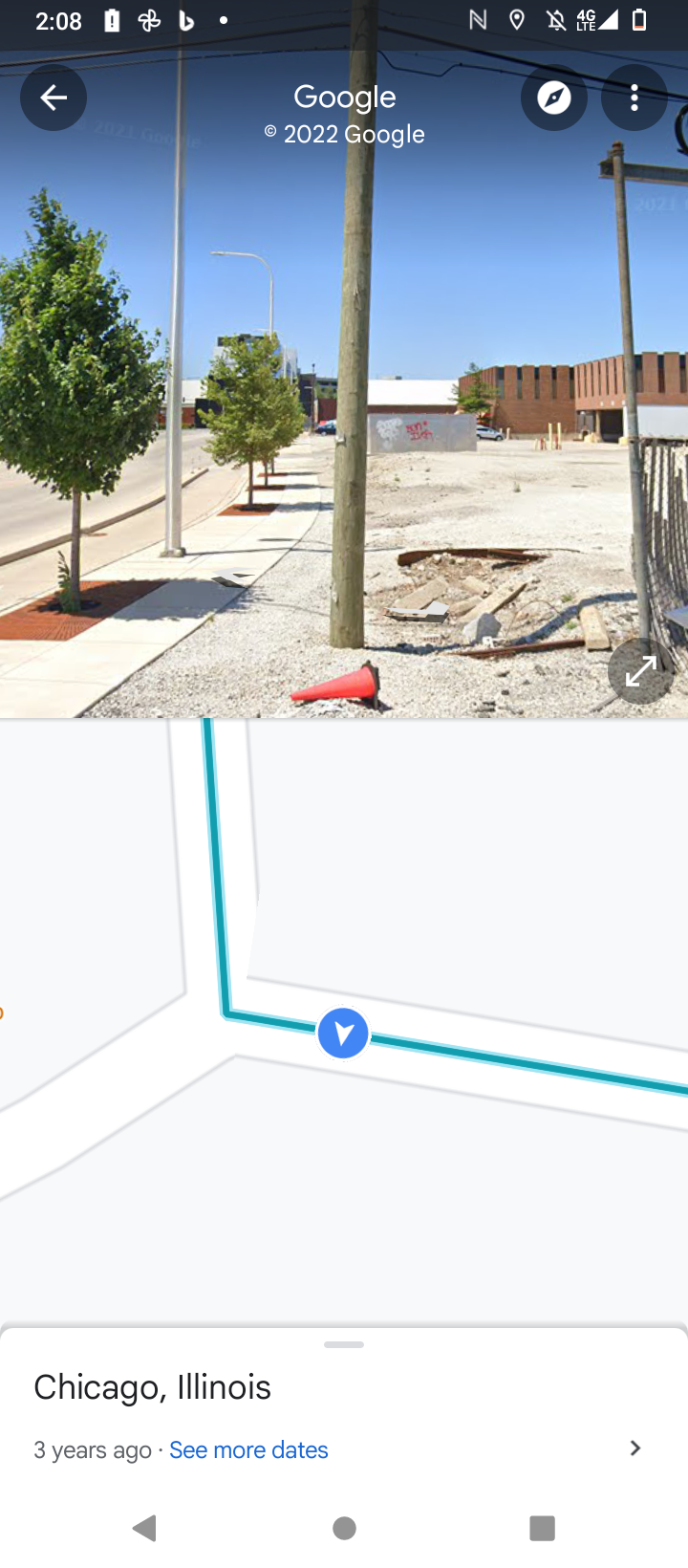The screenshot, taken from a mobile phone, captures a detailed Google Maps interface. The top shows a typical smartphone status bar with the battery almost depleted, 4G signal, and notifications turned off, indicating it is 2:08. Below this, the Google Maps interface, timestamped with "Google 2022 Google" in white text, is displayed. The top half of the screen shows a portrait-oriented Street View image depicting a curved street. The scene is dominated by a blue sky, brick buildings, and a brown telephone pole standing near a patch of torn-up asphalt in what appears to be a damaged or under-construction parking lot. There's a reddish traffic cone tipped over next to the pole, a grey utility cart, silver streetlights, and small trees planted along the pavement. A distant brown brick building and a graffiti-marked dumpster are also visible. Below this Street View is a 2D map section, featuring a Y-intersection with a blue directional arrow pointing from the location depicted above. The map text indicates "Chicago, Illinois," with a note that the view is from three years ago. At the very bottom, there are standard navigation icons: a back arrow, a circle, and a square, alongside a "See more dates" blue link.